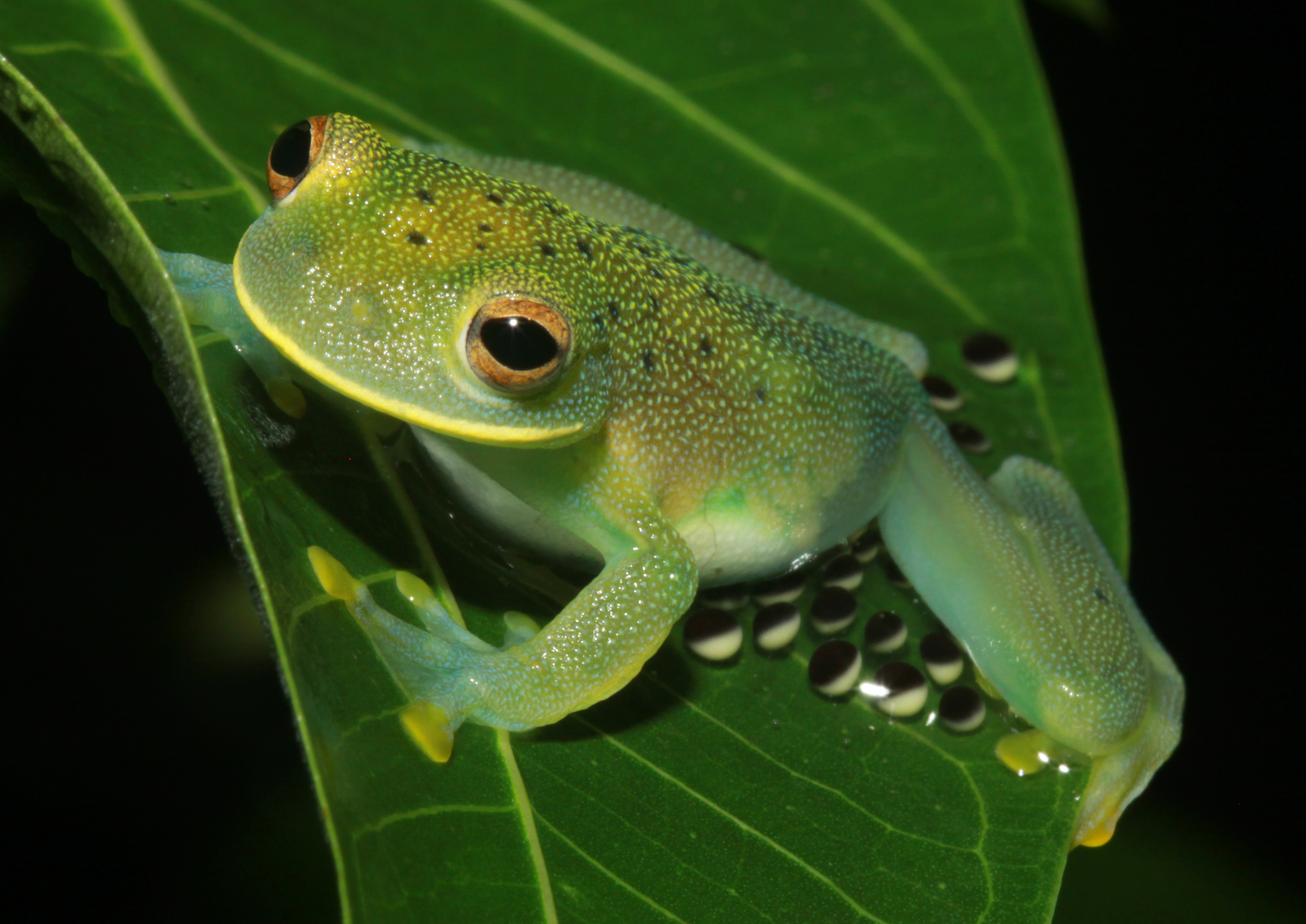The close-up image features a vibrant green frog perched on a similarly vibrant green leaf with intricate light green veins. The frog, likely a tropical tree frog and possibly poisonous, has bright orange eyes with black, beady pupils. Its body is oriented crosswise on the leaf, with its almost flat hands stuck to the surface. Yellow speckles and a distinctive yellow line run across the frog's mouth and head. Below the frog, scattered on the leaf, are disc-shaped objects, probably eggs, that exhibit two colors: black on top and gray or white underneath, with the black portion being more dominant. These dual-colored discs add an intriguing element to the image, hinting at the frog’s reproductive behavior.